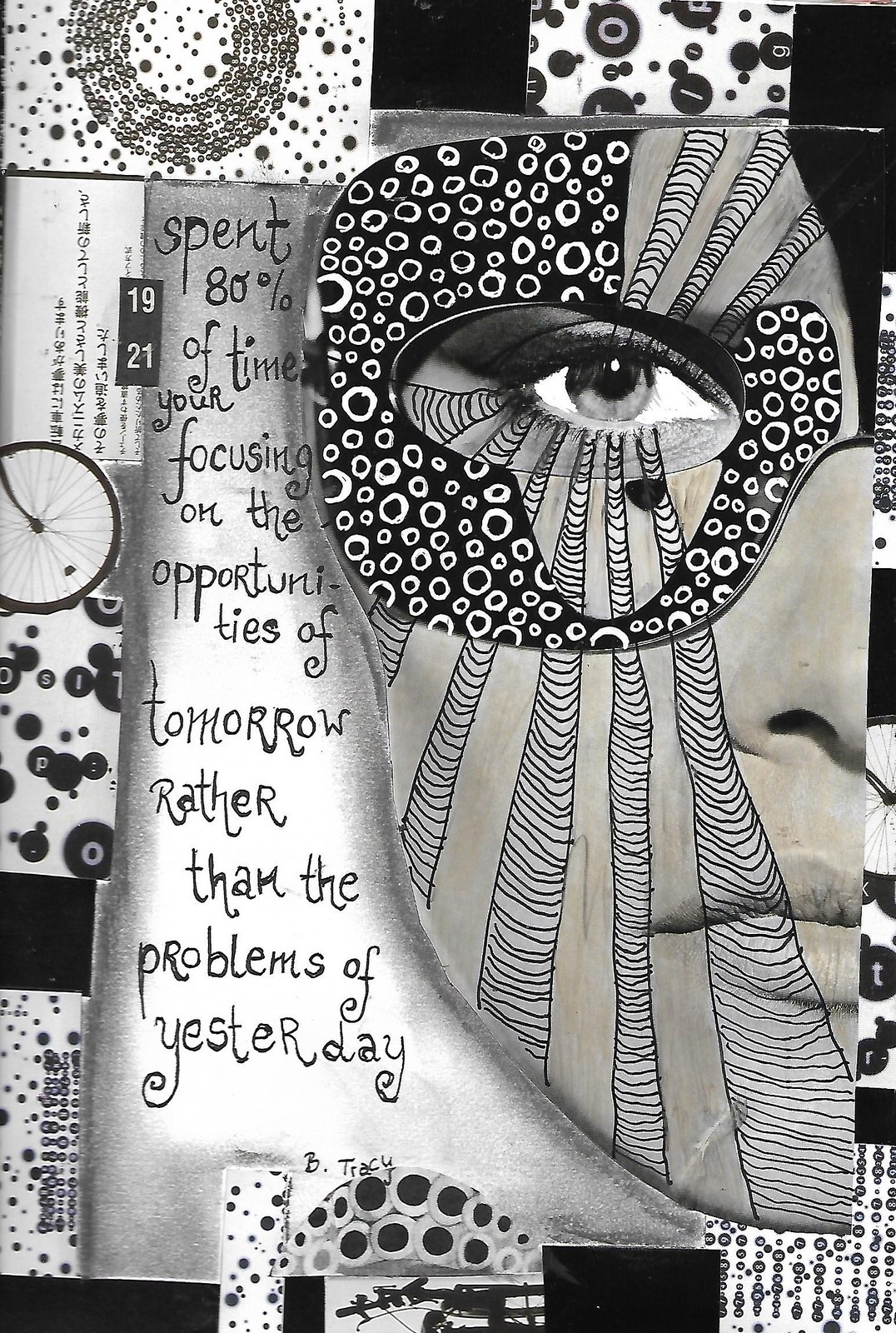This is an abstract, black-and-white collage featuring an intricately detailed half-mask of a woman's face positioned on the right side. The face appears to be made from cloth and displays realistic features, including the left eye, half a nose, and half a mouth. Hand-drawn lines radiate from the eye in various angles, surrounded by small circles. Above the face, there is a strip of material adorned with dots and black circles. The left side of the image includes a piece of paper with the text, "spend 80% of your time focusing on the opportunities of tomorrow rather than the problems of yesterday," with "Be Tracy" written below. Adjacent to the text, there are whimsical designs, including what resembles a turtle shell with dots, a lemon slice, and additional abstract drawings featuring black dots and circles. The overall composition includes elements like bubble designs, Japanese kanji, and floating letters, contributing to the artwork’s dynamic and eclectic presentation.